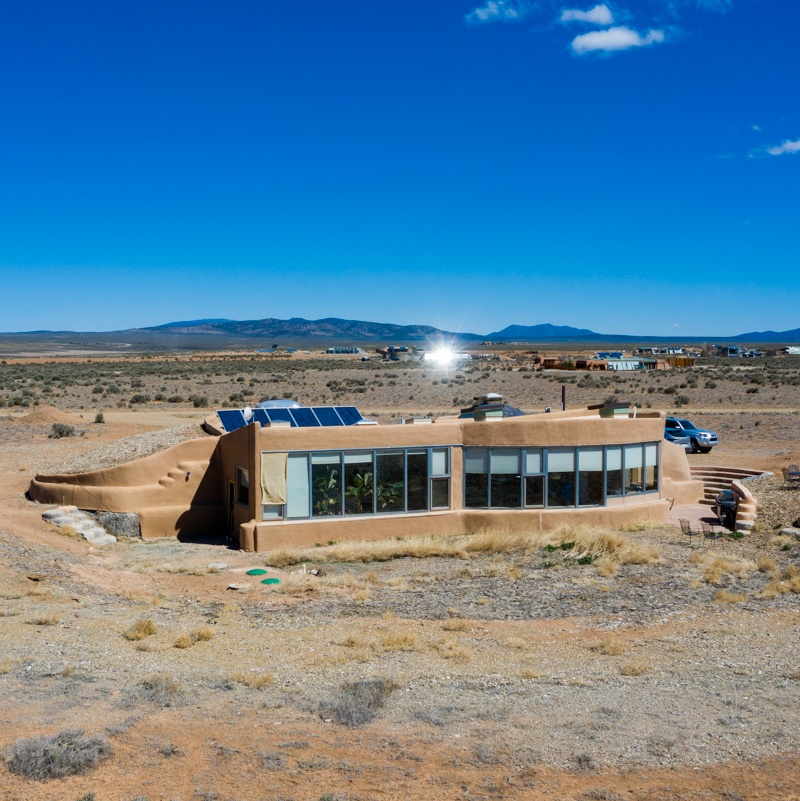In the desert setting, a contemporary, eco-friendly, single-storey home with large floor-to-ceiling bay windows dominates the scene. The house's modern architecture features a curved front wall with extensive windows and a front door, all shaded by pull-down blinds, some of which are partially drawn. The roof, equipped with solar panels, highlights the sustainable design of the structure, which appears to be partially buried, blending seamlessly into the surrounding arid landscape. Round steps encompass the back of the property, leading down to a small sunken patio accompanied by a couple of chairs and minimal greenery visible through the windows. The terrain in front sports a gradient of desert soil colors ranging from dark brown to light gray, yellow, and pale brown, creating an arching pattern in the dirt. In the background, a truck is parked, and a dirt road winds through, leading to other similar residential buildings of what seems to be an eco-friendly housing development. The expansive horizon features distant islands and a relatively low mountain range, under a crystal blue sky with very few clouds.